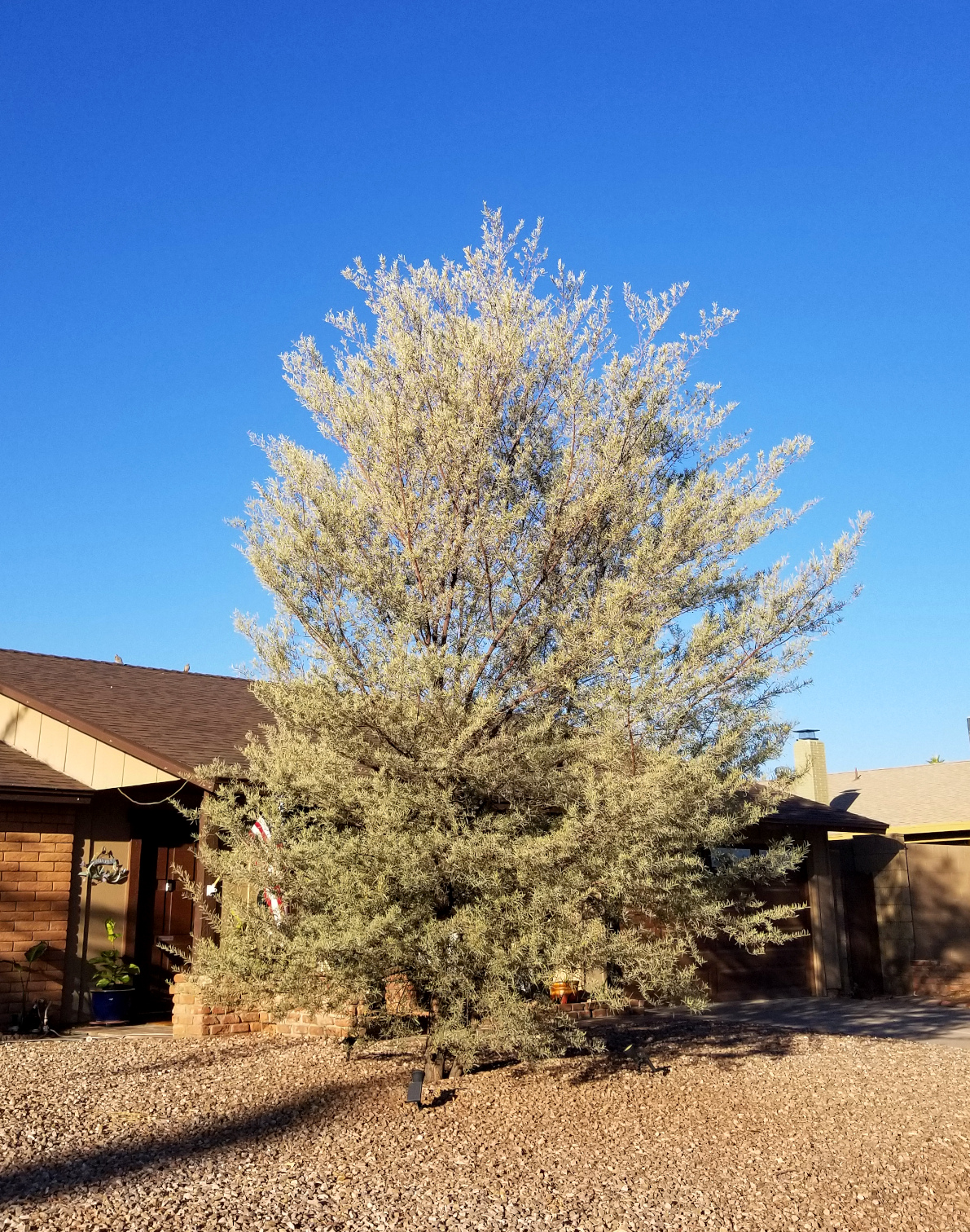The image showcases the front view of a one-story, Rambler-style brick house. The front yard is landscaped with brown and gray gravel, devoid of any green grass. Dominating the scene is a tall, light green tree with thin branches adorned with needles, resembling an evergreen, which allows visibility through its sparse foliage. The house has a dark-colored front door, accentuated by a pot holding a plant next to it. An American flag hangs from a post near the entrance. To the immediate side of the house is a cinder block wall, which serves as a fence separating this property from a similar adjacent house. A paved driveway leads up to the garage. The architectural style and landscaping suggest a location typical of New Mexico, Arizona, or parts of Southern California.